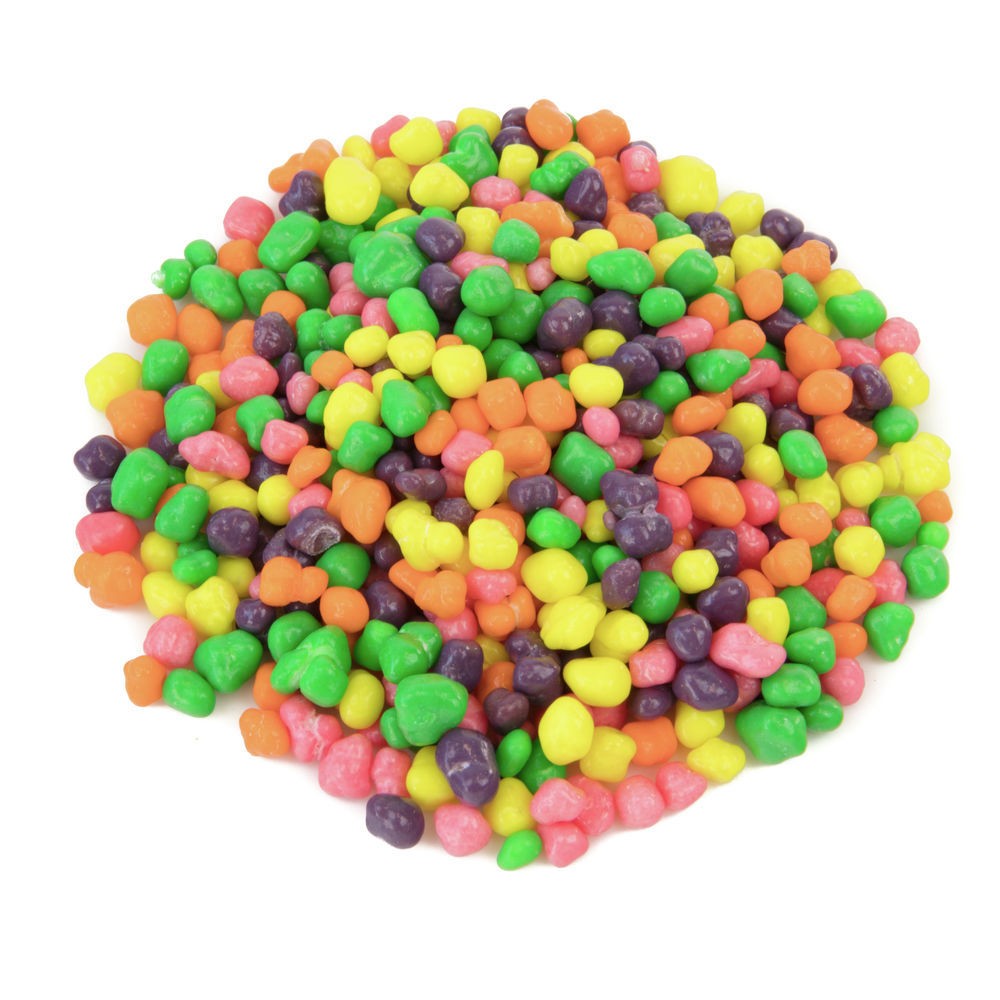The photograph is a close-up shot depicting a pile of colorful Nerds Cluster candy on a plain white background. The candies are small and irregularly shaped, with a lumpy, oblong appearance rather than being perfectly circular. The assortment features a multitude of vibrant colors including yellow, orange, pink, dark purple, and green, all intermixed rather than sorted. The pile is roughly the size of a person's palm, with individual candies being approximately a third the size of a fingernail. The candies are scattered in a way that suggests they've been casually gathered together, forming a mound at the center of the image. The composition highlights the varied textures and shades of the hard candies, some of which appear to be slightly broken or clustered together.